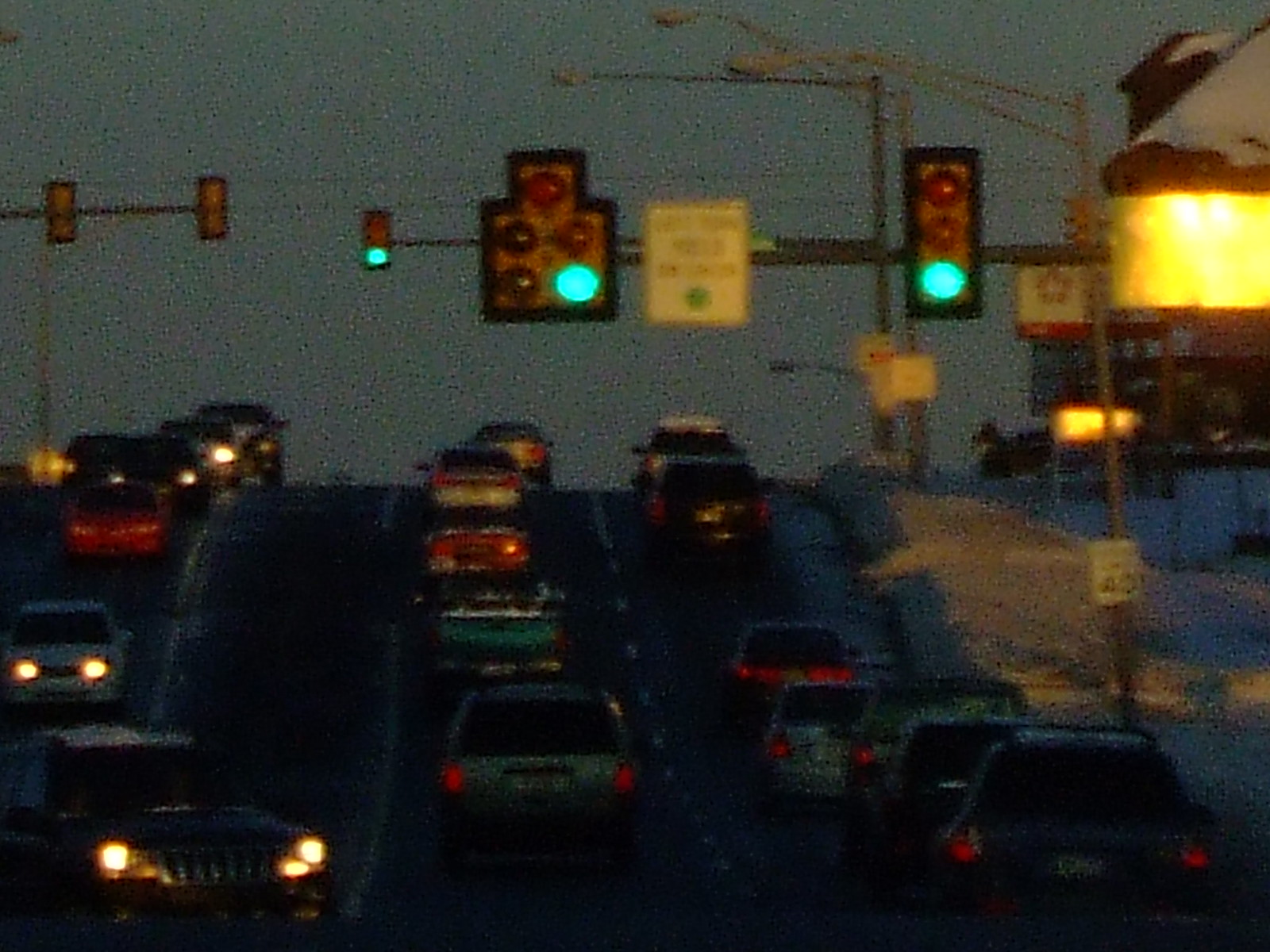A bustling highway is pictured during the evening, likely capturing the rush hour commute. The road, marked with a speed limit sign of 40 miles per hour, features four lanes, packed with a diverse array of vehicles including a blue minivan, a red car, and a green truck. The traffic flows steadily under the guidance of a green traffic light. A central intersection is visible, where a jeep is poised to make a turn. On either side of the highway, signs indicate the presence of a gas station and convenience stores. The roadway, which inclines steeply upward, reveals cars climbing the hill on one side, while cars on the other side descend towards the intersection, all illuminated by the warm glow of the setting sun.